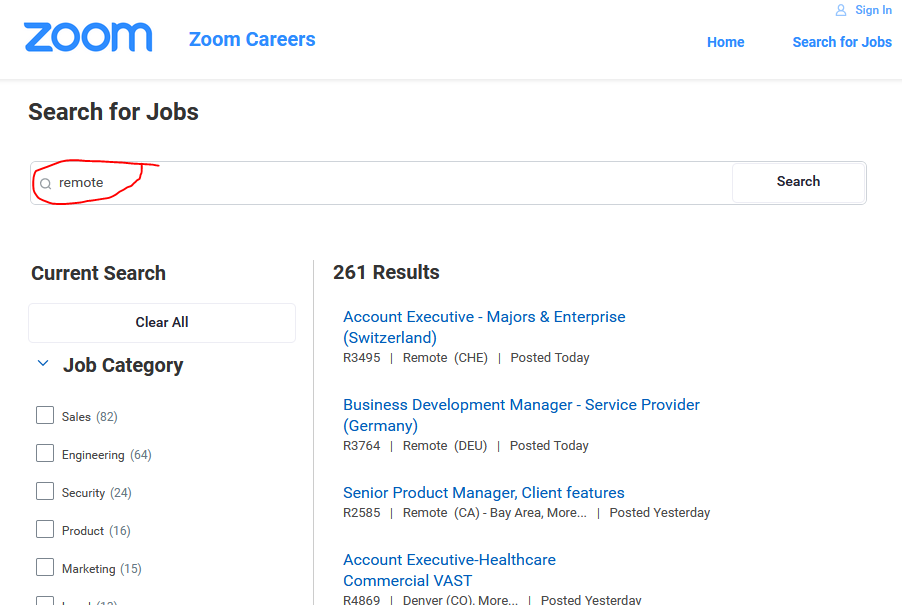The image depicts a webpage with a white background for Zoom Careers. In the top left corner is the Zoom logo in large blue letters, next to "Zoom Careers." On the top right, there's a sign-in button accompanied by a small person icon.

Below the top navigation, a horizontal menu includes "Home," a vertical separator line, followed by "Search for Jobs." Underneath this menu, there is a search bar with a magnifying glass icon on the left side. Inside the search bar, the word "remote" is encircled in red, and there is a white 'Search' button to its right.

The page is segmented into two sections. The left section is titled "Current Search," featuring a 'Clear All' button beneath it. Below this button, there is a "Job Category" section listing several job categories, each accompanied by a corresponding number in parentheses and an empty checkbox:

1. Sales (82)
2. Engineering (64)
3. Security (24)
4. Product (16)
5. Marketing (15)

To the right, the search results section displays "261 results" in bold black text. The results include:

1. **Account Executive - Majors & Enterprise (Switzerland)**  
   Code: R3-R3495  
   Status: Remote (CHE)  
   Posted: Today

2. **Business Development Manager - Service Provider (Germany)**  
   Code: R3764  
   Status: Remote (DEU)  
   Posted: Today

3. **Senior Product Manager, Client Features**  
   Code: R2585  
   Status: Remote (CA - Bay Area)  
   Additional Info: more...  
   Posted: Yesterday

4. **Account Executive - Healthcare, Commercial VAST**  
   Code: R4869  
   Location: Denver, CO  
   Additional Info: more...  
   Posted: Yesterday

The layout is structured and clearly delineates navigation, search options, job categories, and detailed job listings.